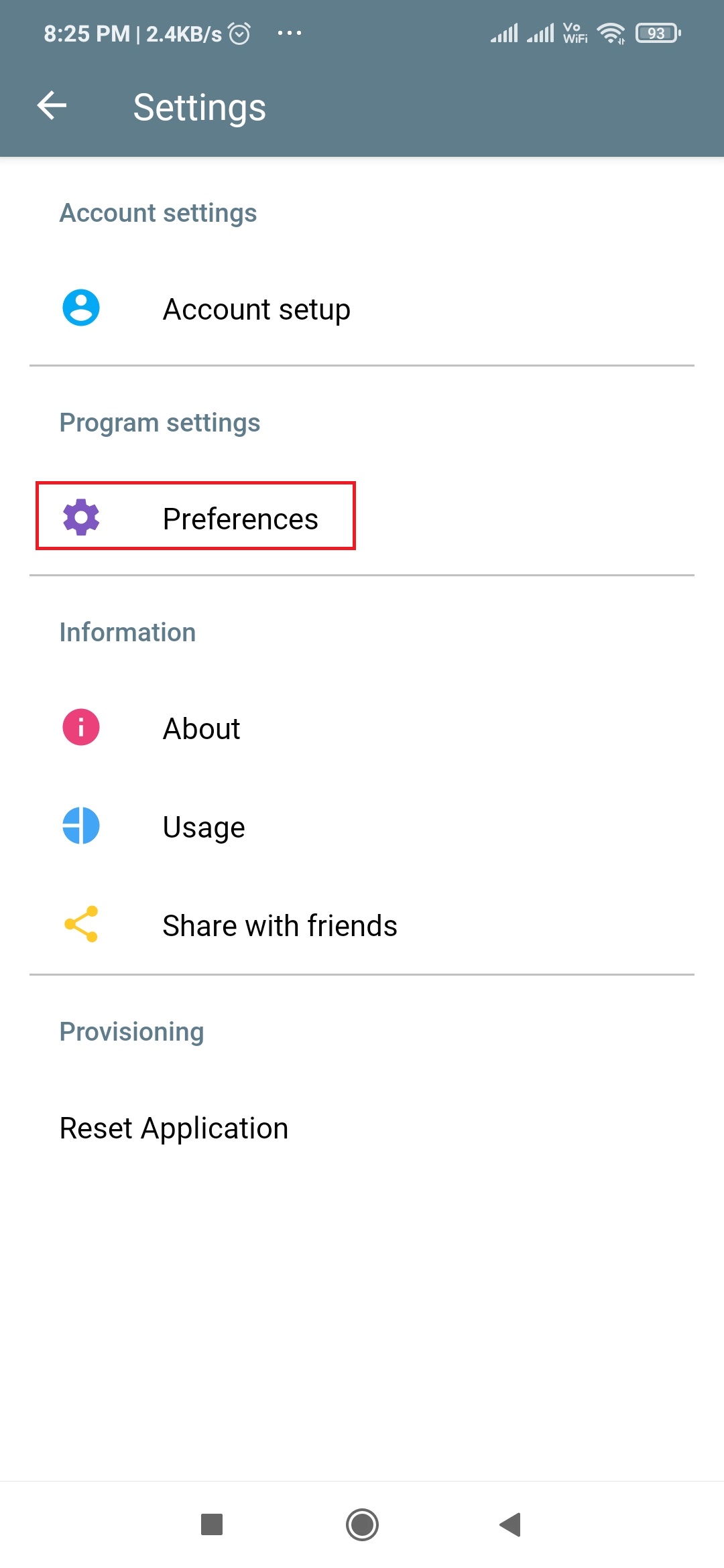This is a detailed screenshot of an app's settings page. At the top, there's a gray header with a back arrow and the word "Settings." The first section, labeled "Account Settings," features an item called "Account Setup" accompanied by a default blue avatar icon. Below this is a line divider.

The next section is labeled "Program Settings" and includes an item named "Preference," which is highlighted with a red rectangle and features a purple gear icon. Another line divider follows.

The subsequent section is "Information," containing three items: "About," "Usage," and "Share with Friends." The "About" item has a red circle with a white eye icon, "Usage" displays a blue circle segmented into one half and two quarters, and "Share with Friends" features a share icon made up of three connected yellow dots.

The final section appears to be repetitive and unclear. It mentions sharing multiple times but continues to describe sharing with friends. A red triangle, cut off in the middle, is also mentioned but its exact location and purpose are unclear.